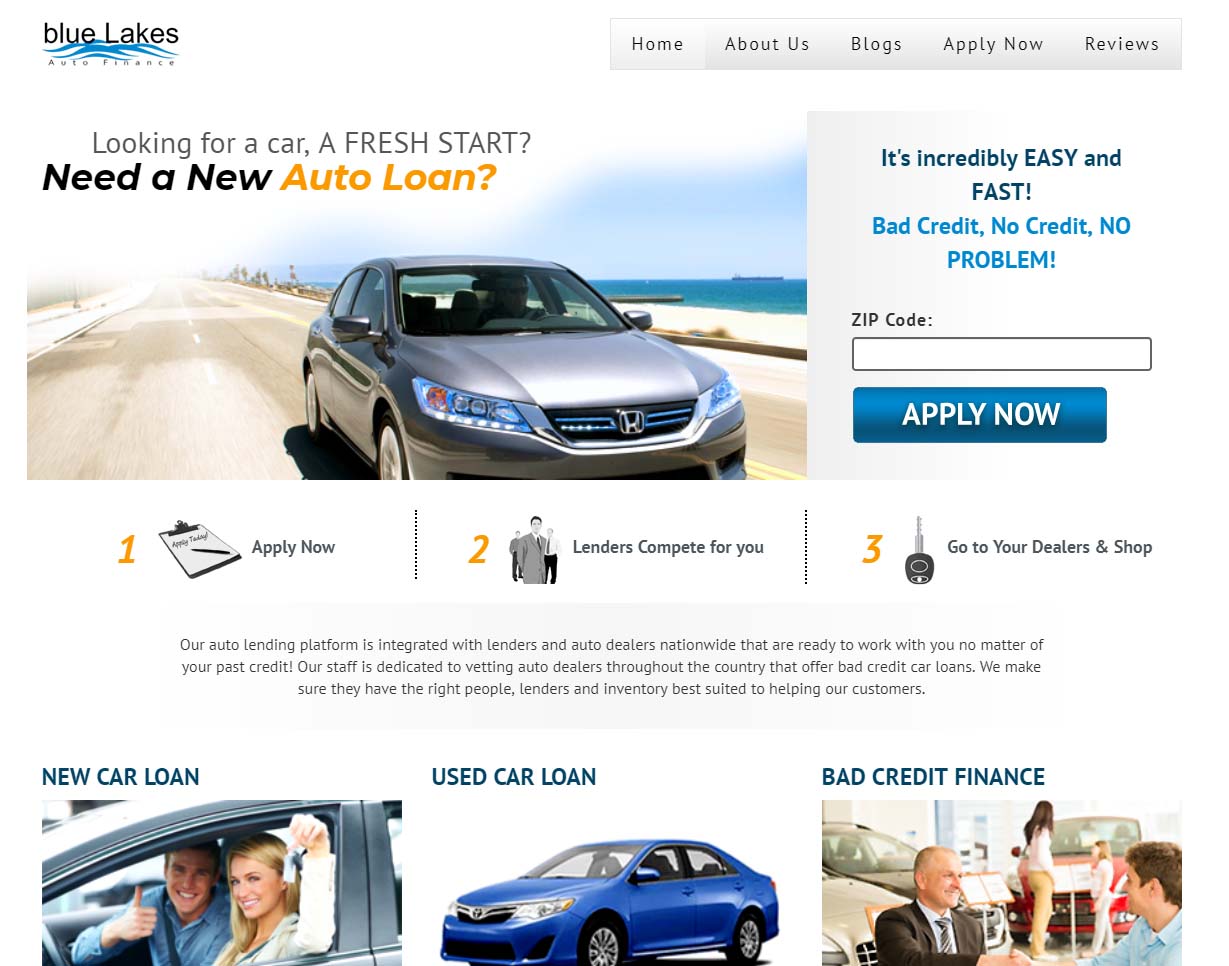The image is a screenshot of a website for "Blue Lakes Auto Finance," a company providing auto loans. The logo, located in the upper left corner, features the company name "Blue Lakes" written in dark gray, lowercase letters, accompanied by stylized blue wave motifs symbolizing water. Just beneath the company name, in smaller gray font, is the tagline "auto finance."

The top menu bar has a white background, transitioning to a very light silver-gray on the right side where navigation items are listed in gray font. From left to right, the menu options are: "home," "about us," "blogs," "apply now," and "reviews."


Near the top left of the page, there's an image of the front part of a silver car with a scenic background likely depicting a lake, in line with the company's theme. Dominating the central portion of the screen, a headline poses the question, "Looking for a car a fresh start?" Following this, in bold black letters, it states "Need a new" with "auto loan?" highlighted in gold.


On the right side of the page, set against a gray background, a promotional message reads, "It's incredibly easy and fast," followed by a sky-blue phrase, "Bad credit? No credit? NO PROBLEM!" emphasized in capital letters and an exclamation mark. Below this, a rectangular input field labeled "zip code" allows users to enter their zip code, followed by a blue rectangular button with "apply now" in white font.

Further down, the site outlines its simplified loan application process in three steps:
1. "Apply Now."
2. "Lenders Compete for You."
3. "Go to Your Dealers and Shop."

At the bottom of the page, there are three sections, each highlighting different auto loan services. The first section, titled "New Car Loan," shows a happy couple — a smiling woman in the driver's seat holding car keys, and a man beside her giving a thumbs up. Both individuals appear to be white. The middle section, "Used Car Loan," displays a side view of a blue sedan. The final section, "Bad Credit Finance," features an image of two men, one in a brown suit and the other in a light blue shirt, shaking hands, both appearing to be white.